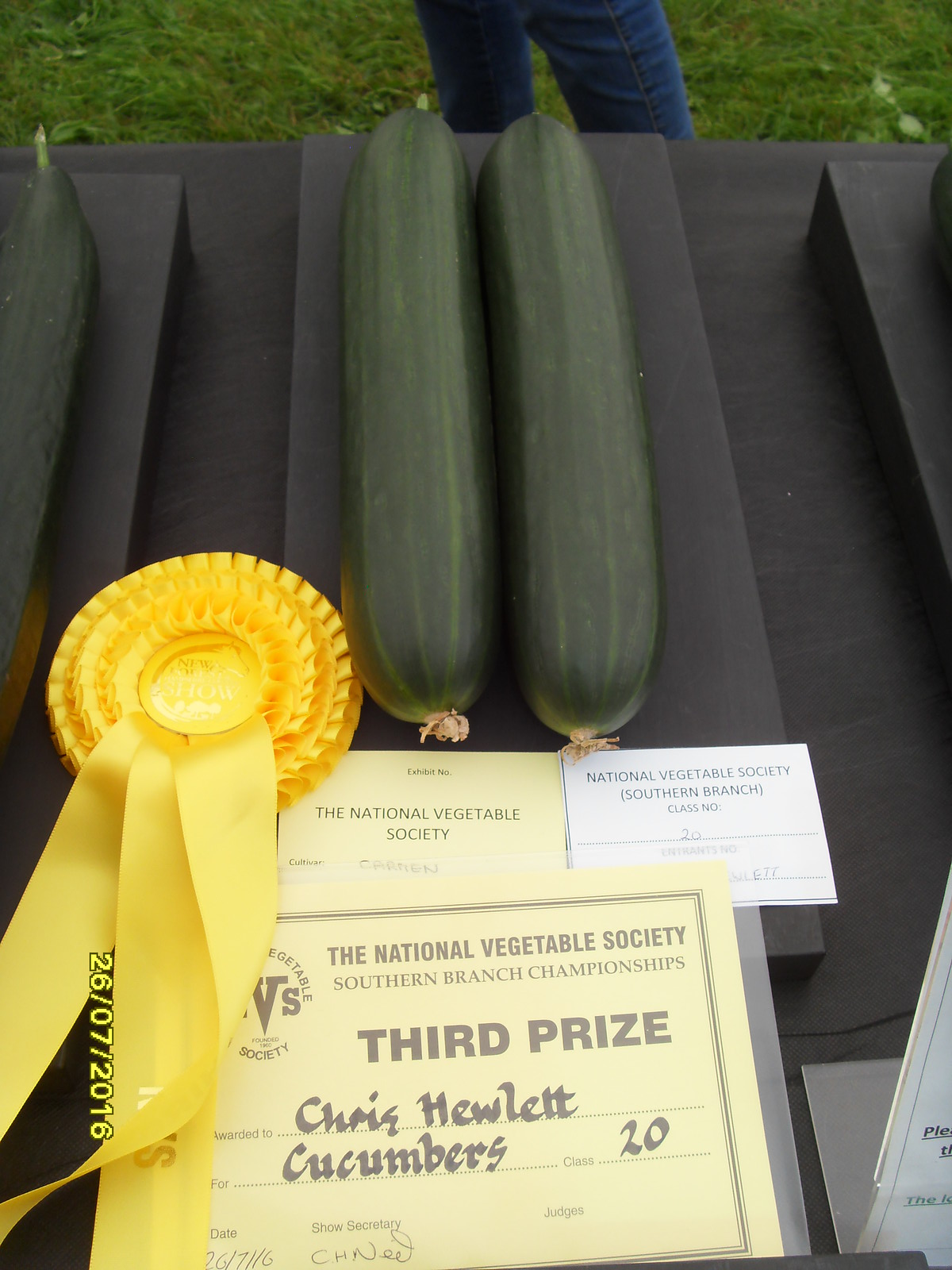The image is an outdoor photograph taken during the daytime, showcasing an entry in a vegetable contest. The focal point is a black table covered with a black tablecloth, on which three rectangular black boxes are placed. Each box holds large, perfect cucumbers. The central box, which is fully visible, contains two cucumbers and is narrower compared to the ones partially visible on the left and right of the frame.

Several signs and cards are positioned around the cucumbers. On the left, a card with a light yellow background and black print identifies the exhibit as belonging to the National Vegetable Society and lists the cultivar as Cartien. Another sign to the right announces the National Vegetable Society, Southern Branch, class number 20.

A prominent yellow ribbon placed to the left of the cucumbers signifies a third-place award. Below this ribbon is a larger certificate declaring that Chris Hewlett has been awarded third prize at the National Vegetable Society, Southern Branch Championships for cucumbers in class 20. The certificate is dated 26-07-2016.

At the top edge of the image, a strip of grass on the ground is visible along with a person’s legs, clad in blue jeans, framing the scene and hinting at the outdoor setting of this vegetable competition.